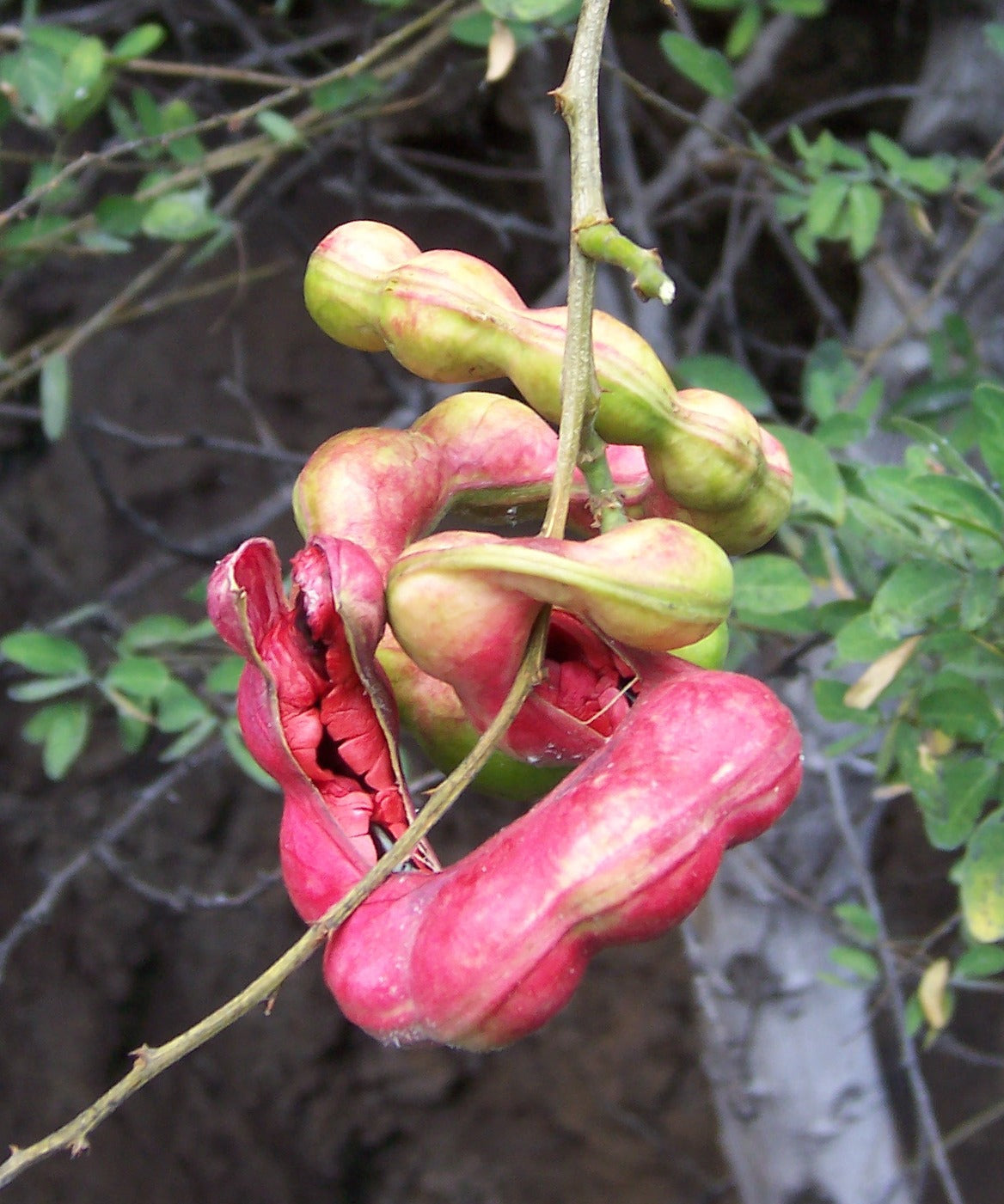The image is a close-up of an unusual plant with legume-like pods attached to a coiling green stem that runs from the top center to the lower right, curving as it descends. The pods, resembling elongated peanut shells, are in various stages of ripeness and color. The topmost pod is predominantly olive green, while the central one has a mix of green and rosy tinges. The bottom pod, distinctly crooked and split open, reveals pinkish-red hues with visible flower petals inside. These pods cascade around the stem in a spiral pattern, creating a visually striking arrangement. In the background, a chain link fence and an assortment of green foliage, along with crisscrossing branches and a gray tree trunk, add depth and texture to the scene.